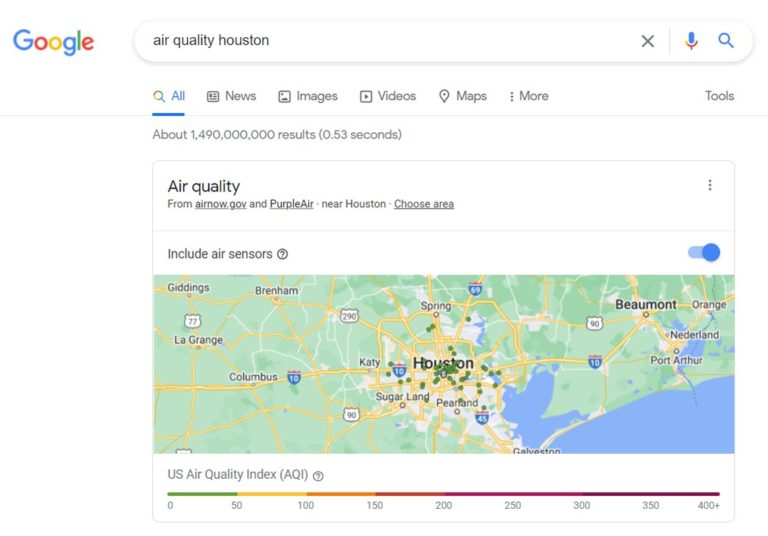The image features a screenshot of a Google search page with a white background and thin blue lines framing the content. In the top left corner, the Google logo appears in its signature colors of blue, red, yellow, and green. Below the logo, the search query entered is "air quality Houston," which is highlighted and underlined in blue.

Just beneath the search bar, there is a navigation menu offering various categories such as "All," "News," "Images," "Videos," "Maps," and "More." On the far right, there is an option labeled "Tools." The search results indicate approximately 1,490,000,000 results generated in 0.53 seconds.

Following a dividing line, the first entry presents information sourced from "AirNow.gov" and "PurpleAir," focused on air quality in the Houston area. A blue slider button, represented by a large circle, is included in this section.

The image also contains a detailed map showcasing the air quality index (AQI) for various regions within and around Houston, including Beaumont. The AQI scale, ranging from 0 to 400+, is accompanied by a circle with a question mark, presumably for additional information or definitions regarding the air quality index.

This detailed visual provides a comprehensive overview of current air quality metrics, emphasizing Houston's environmental conditions as assessed by reliable sources.